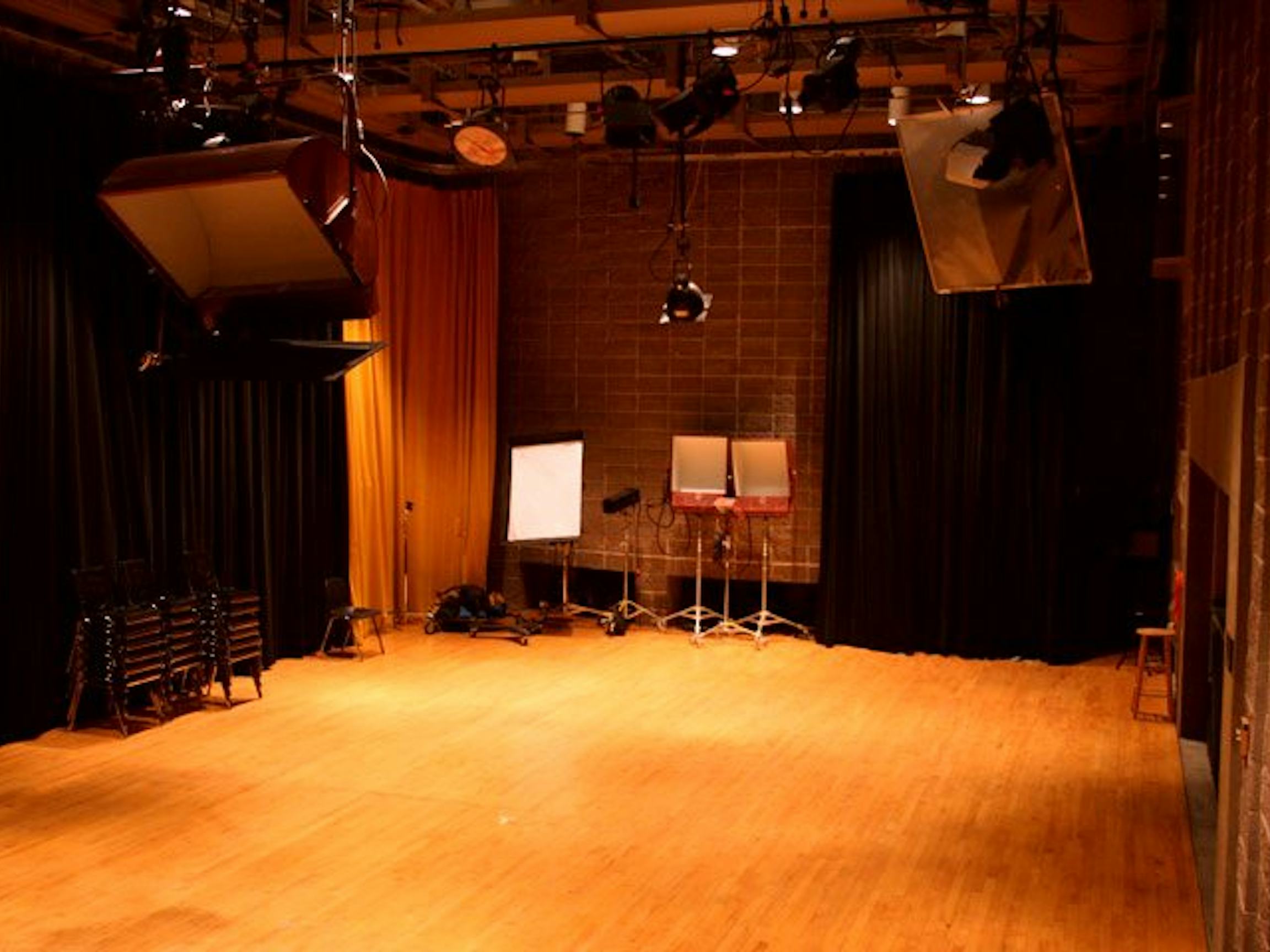This is a detailed color photograph depicting a large, empty indoor room, possibly a musical studio or stage. Despite the overall blur, several distinct features are notable. The ceiling is adorned with multiple light fixtures, including half a dozen small lights and a few large box lights, some of which are lit while others are not. The backdrop is a striking red brick wall, partially covered by a large black curtain that extends from the ceiling to the floor. On the left side, the scene is framed by another black curtain with a yellow curtain adjacent to it. In front of these curtains, three stacks of black chairs are neatly arranged, with an additional single chair visible in the background. Moreover, several light stands are positioned in front of the brick wall, contributing to the room’s stage-like ambiance.